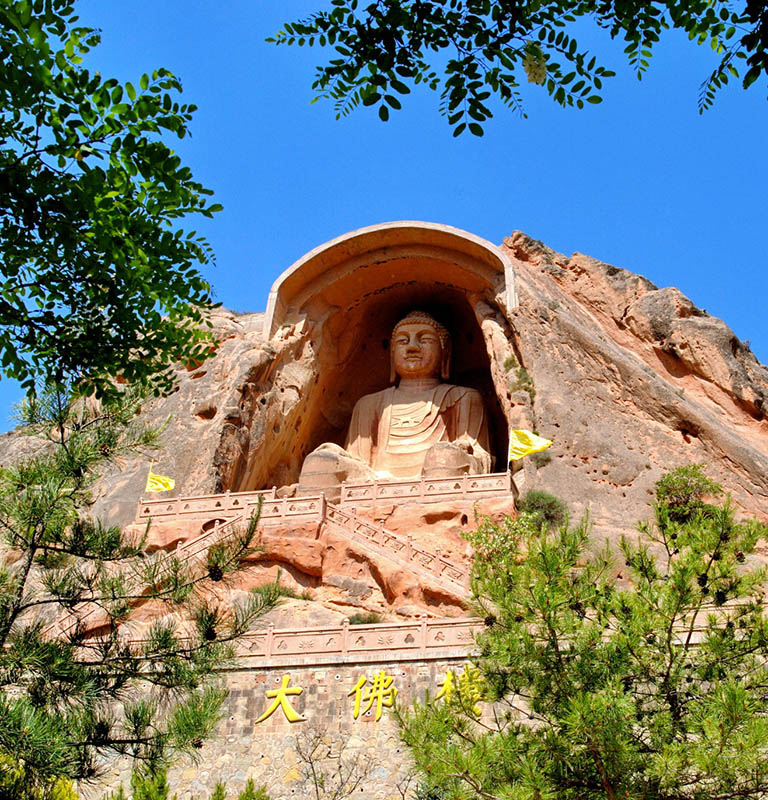The image is a vertical photo that captures a large rock or mountain with a detailed, intricately carved statue. The carved figure appears to be a man or deity, seated with visible knees, chest, and face, adorned with what looks like a crown of braided hair or a head covering. The figure is enrobed in garments that feature intricate patterns. This statue is part of a larger architectural carving that includes stairs, a balcony terrace, and other detailed ornamental elements, giving the appearance of a temple structure. Below the statue, near the bottom of the rock, are three yellow Asian symbols, likely Chinese or Mandarin characters. The scene is framed by a brilliant light blue sky above, with green fronds and tree branches, some resembling pine needles, extending into the frame. Fruits can be seen hanging from the trees that flank the rocky hill. The perspective suggests the photo was taken from the ground, looking up at the awe-inspiring structure.